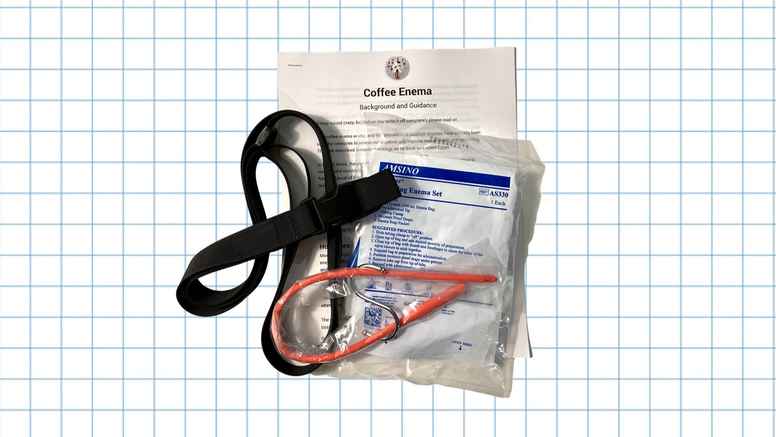The image depicts a disconcerting product set against a background reminiscent of blue-lined graph paper, dividing the scene into small white squares. Centrally positioned are several objects frequently associated with medical procedures. At the top of an instructional booklet titled "Coffee Enema: Background and Guidance," a series of stapled papers provide detailed yet unreadable instructions. Resting haphazardly on these documents is a black strap or belt, adding an element of uncertainty. To its right, a clear plastic bag with obscure blue lettering contains an orange-colored tube and a silver S-clamp, evocative of an IV setup. The intricate details of the plastic packaging and associated components make the image particularly unsettling.